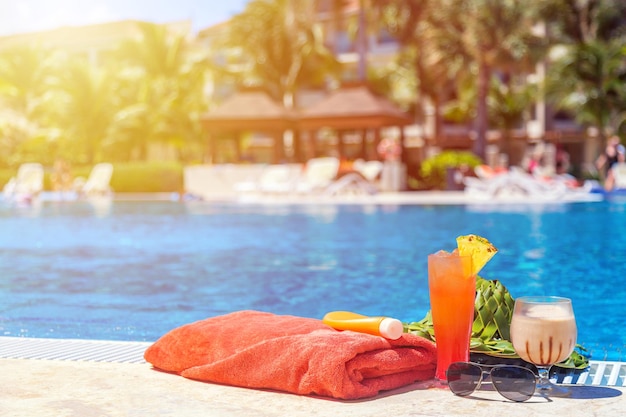In the bright glare of the sun, the photograph captures a serene, sun-soaked afternoon at what appears to be a resort or club. The vivid blue pool dominates the background, with gentle water ripples and blurred images of palm trees, lounge chairs, and possibly a hotel structure. The focus, however, rests on the foreground, where an inviting scene is meticulously detailed. A rolled-up reddish-orange towel lays on the concrete by the poolside, topped with an orange bottle of sunscreen with a white lid. A tall, clear glass holds a vibrant mixed drink, transitioning in color from red at the base to orange at the top, garnished with a slice of pineapple. In front of the glass, a pair of aviator sunglasses shines in the sunlight, their reflective lenses adding a chic touch. To the right, another drink, presumably a smoothie, rests inside a wide circular cup with a pinkish, creamy liquid. A woven green sun hat completes the arrangement, hinting at leisurely, sun-filled relaxation. The overall composition evokes a peaceful and enjoyable sunny day at a luxurious resort.